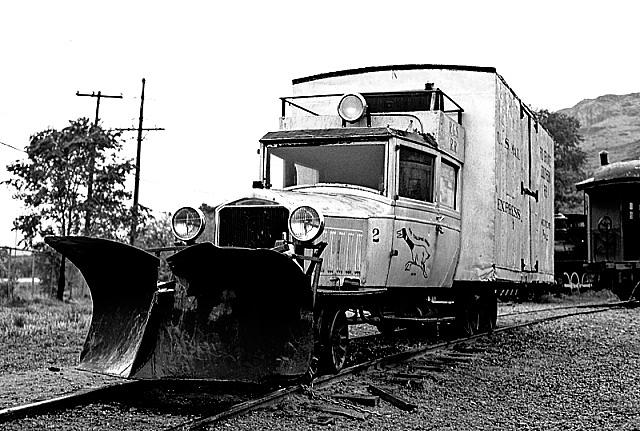This black and white photograph, likely from the 1920s or 1930s, depicts a vintage utility truck with train-like wheels perched on old, worn railroad tracks. The sky in the image is a stark white, enhancing the age-old ambience of the scene. The truck, which appears to be light-colored, possibly white, features a large container section at the back, reminiscent of a delivery or freezer truck. Its front is equipped with a dark metallic plow or scoop, suggestive of a device used to clear dirt, debris, or snow, flanked by two prominent headlights.

To the left of the truck, several telephone poles and a tree frame the scene, with additional vegetation visible in the distance, creating a relatively flat landscape. Behind the truck, the railroad tracks reveal more vintage elements: an old, dark-colored train car followed by what seems to be a steam locomotive, suggesting historic industrial activity. A distant hillside completes the background, contributing to the timeless quality of the photograph.